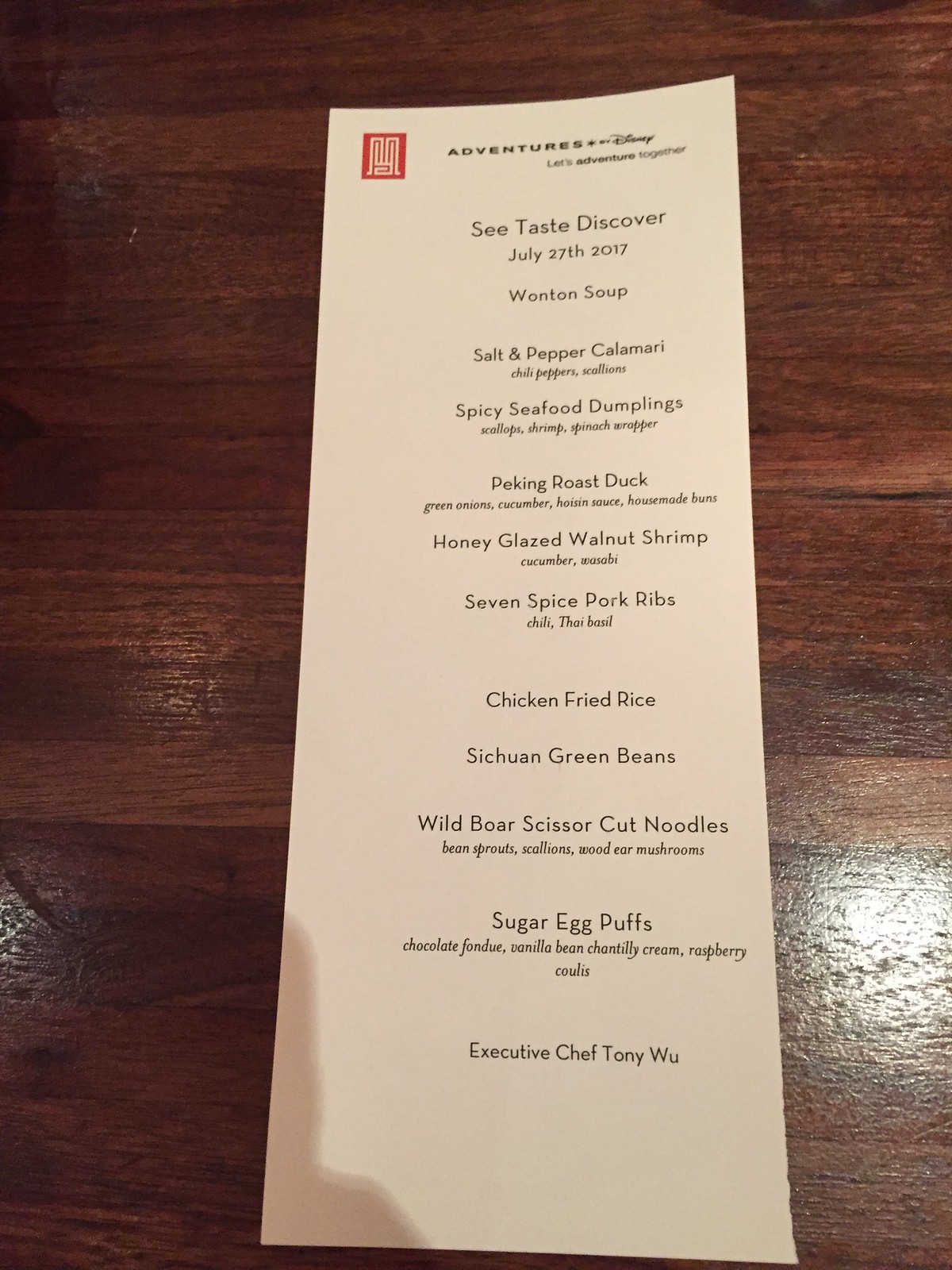The photograph features a detailed menu placed on a well-worn, brown wooden table, showcasing the distinctive grain lines and etchings of the wood. The menu itself is an elongated, rectangular piece, prominently titled "Adventures by Disney" at the top. This title is accompanied by a red emblem with intricate white line designs reminiscent of Aztec patterns.

Below the main heading, the menu invites patrons with the phrase "Let’s Adventure Together," followed by "Sea, Taste, Discover" and the date "July 27th, 2017." The culinary offerings begin with "Wonton Soup," "Salt and Pepper Calamari with Chili Peppers and Scallions," and "Spicy Seafood Dumplings." Although some text below is not legible, "Shrimp" and various other items can be noted, followed by "Spinach," before listing the further detailed:

- "Peking Roast Duck with Green Onions and Cucumber,"
- An illegible dish,
- "Honey Glazed Walnut Shrimp with Cucumber,"
- Another indistinct item,
- "Seven Spice Pork Ribs,"
- "Chili Thai Basil Chicken,"
- "Fried Rice,"
- "Szechuan Green Beans,"
- "Wild Boar Scissor Cut Noodles with Bean Sprouts, Scallions, and Wood Ear Mushrooms."

Dessert selections include "Sugar Egg Puffs," "Chocolate Fondue," "Vanilla Bean Chantilly Cream," and "Raspberry Coulis." The executive chef for this adventurous culinary journey is noted as "Tony Wu."